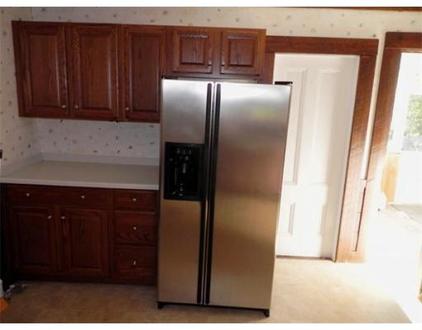This photograph captures a clean, seemingly unoccupied kitchen featuring a prominently positioned stainless steel side-by-side refrigerator. The refrigerator has two handles, with the right side slightly wider than the left, which includes a black ice and water dispenser. Surrounding the refrigerator are dark brown wooden cabinets with white countertops, both to the left and above. The kitchen wall is adorned with white wallpaper decorated with small, somewhat indistinct circular patterns or dots. The floor is a light tan or brown color. 

To the right of the refrigerator, there are two doorways: one with a white door set in a dark brown wooden frame, and the other doorway is open, revealing a glimpse into another room with green leaves visible and light streaming through. Overall, the scene is free from any personal belongings or furnishings, suggesting the house might be unoccupied.